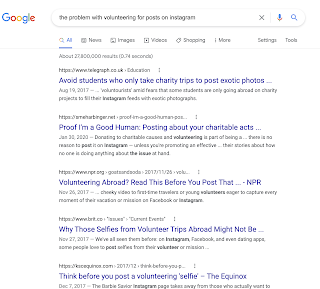The image is a screenshot of a Google search. At the top of the screenshot, the iconic Google logo appears in its distinctive multicolored lettering. Below the search bar, the query entered reads: "the problem with volunteering for post on Instagram." 

Highlighted and underlined in the search bar is the word "awe." The page displays a list of search results, where each result title appears in blue, indicating clickable links. There are five main search outcomes presented:

1. "Avoid students who only take charity trips to post exotic photos."
2. "Proof I'm a good human posting about your charitable acts."
3. "Volunteering Abroad: Read this before you post that."
4. "Why those selfies from volunteer trips abroad might not be..."
5. "Think before you post a volunteering selfie."

The search results include articles emphasizing the importance of genuine charitable acts over self-promotion, and most have publication dates of 2017, except for one result which is dated 2020. One of the articles is noted to come from a source called "The Equinox."

This detailed screenshot captures a critical look at the motivations behind sharing volunteering experiences on social media, encouraging thoughtful reflection on authenticity and the impact of such posts.